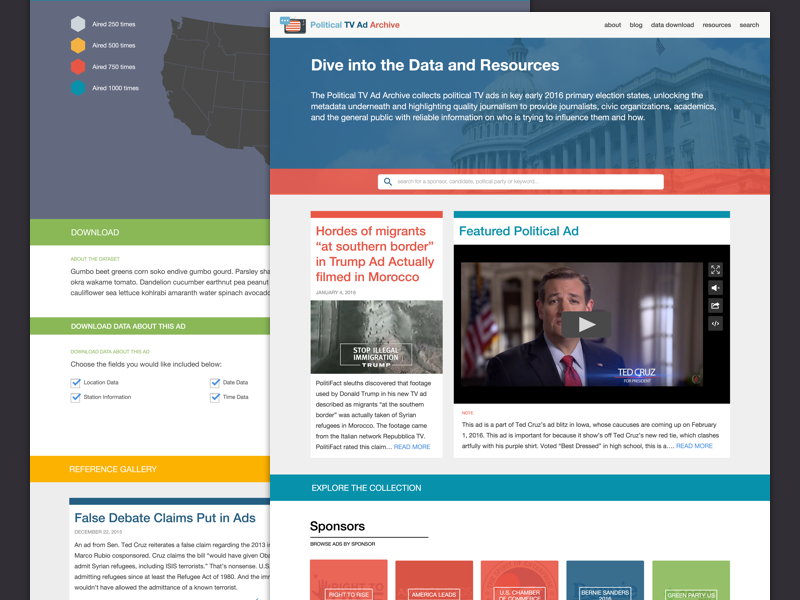The pop-up is vibrant and structured, with distinct sections. The top portion has a white background featuring the text "Political TV" in blue, followed by "Archive" in red. Adjacent to this, in black, it lists navigation options: About, Blog, Data, Download, Resources, and Search. Below, a blue background showcases a filtered image of the White House, giving it a bluish hue. Overlaid in white text, it reads: "Dive into Data and Resources. The Political TV Ad Archive collects political TV ads in early 2016 primary election states, unlocking the metadata underneath and highlighting quality journalism. This provides journalists, civic organizations, academics, and the general public with reliable information on who is trying to influence them and how."

A red border extends horizontally, featuring a white search box with placeholder text in gray that says, "Search for sponsor, candidate, political party, or keyword." Beneath this section, a video thumbnail displays with a gray pause button overlay. Ted Cruz is visible in the thumbnail, wearing a red tie and black blazer, with an American flag in the background. Teal text denotes this as a "Featured Political Ad."

To the side, red text highlights: "Hordes of Migrants at Southern Border and Trump Ad Actually Filmed in Morocco." A green border below this section contains the text "Download" in white, followed by another green border with "Download Data About This Ad" in white. An orange border with white text reads "Reference Gallery." Finally, at the bottom of the page, a blue headline states: "Forced Debate Claims Puts in Ads."